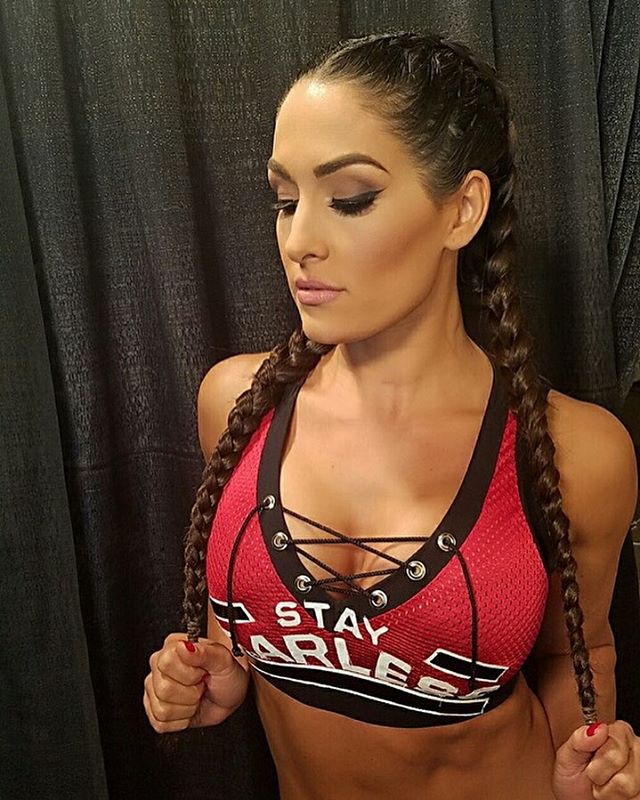This color photograph showcases Nikki Bella, a female athlete and wrestler from the United States, standing in front of a black curtain. She has long brown hair styled into two braids, one on each side, which she is holding with her hands. Nikki is posed looking down, revealing her eye makeup consisting of brown smokey eye shadow and black eyeliner. Her lips are adorned with pale pink lipstick. She wears a red and black athletic sports bra with lace-up straps, featuring the partially visible text "STAY A R L E". The red and black theme extends to her red nail polish, matching her sports bra. Her attire exposes her midriff, neck, shoulders, and a hint of cleavage. The lighting emphasizes Nikki's face, making her the focal point against the dark background.